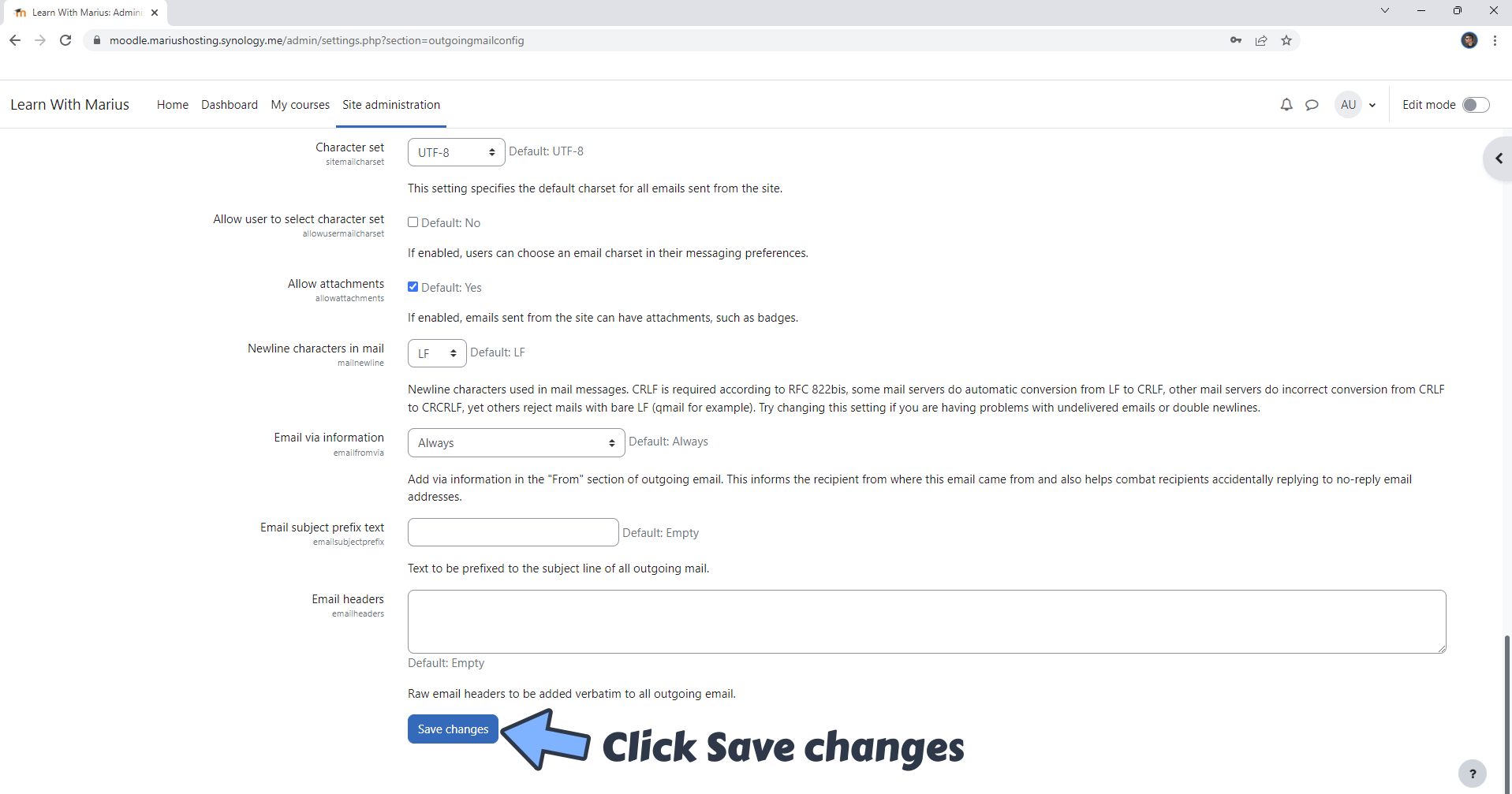**Caption for the Image:**

The image displays a screenshot of the "Learn with Marius" interface, situated at the top-left corner, against a gray bar that includes various control elements like a dropdown menu, and minimize, maximize, and close buttons. Below these controls, there is a detailed section of settings for email configuration within the Moodle platform hosted by Marius on Synology.

The first setting line reads "Moodle.marius.hosting.synology.me/user". This section includes options like:

- **User Email Configuration**: Whether users can choose their email address (default set to 'no').
- **Attachment Permissions**: Option to allow or disallow attachments, enabled by default.
- **Email Formatting and Compliance**: Mentions the use of 'CRLF' (Carriage Return Line Feed) formatting as required by RFC 82BIS standards. It references the conversion of line break formats from 'LRF' to 'CRLF'.
- **Problem Resolution**: Advice is given for situations involving issues with undeleted emails and double new lines, suggesting users refer to additional information for resolving such problems.

Each setting is denoted with checkboxes and default states, ensuring the administrator can customize the email interaction policies to meet compliance and user needs.